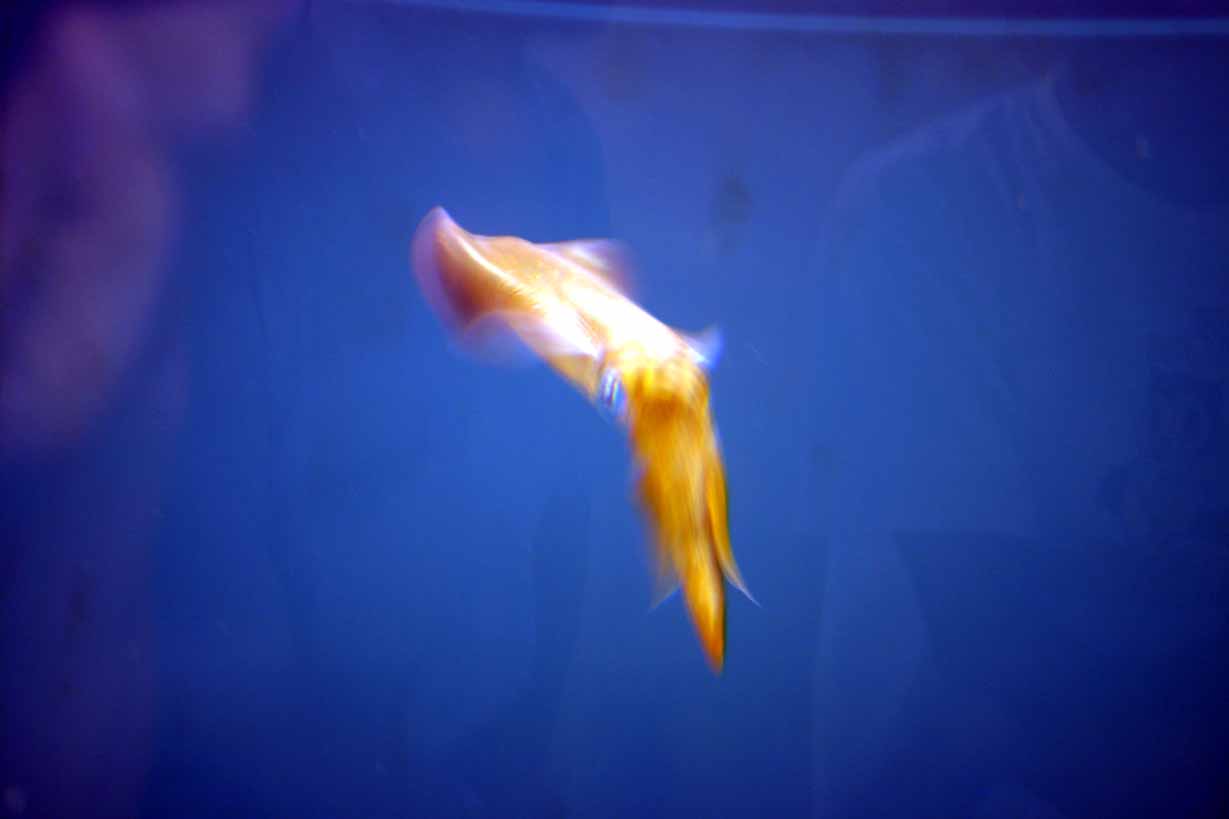The image depicts a scene with a blue background, likely suggesting an underwater environment or an aquarium tank. At the center of the image is a fuzzy and out-of-focus golden and white organism that resembles either a squid or a koi fish, characterized by long, trailing tentacles or tail. The creature appears to have eyes on either side and is slightly blurred, adding to the ambiguity of its exact nature. The glass surface of the tank reflects the figure of a man wearing a white crew neck short-sleeve t-shirt on the right side of the image. This reflection is clear enough to notice the person's attire and position, indicating their proximity to the tank. The overall setting conveys an aquarium-like habitat, filled with water, accentuated by the deep blue hue surrounding the unique marine creature.